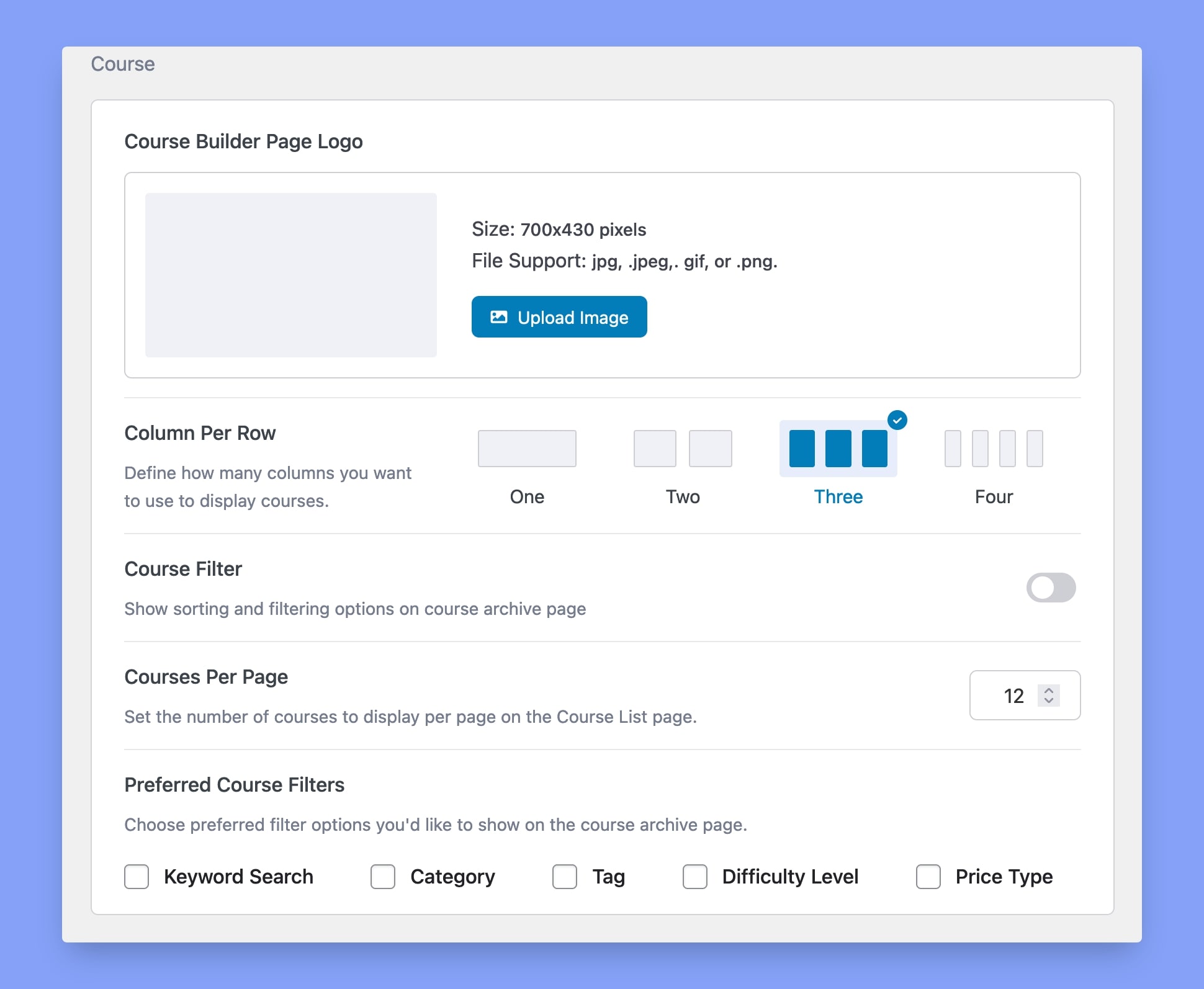This is an image of a course management page. At the top left corner, the word "Course" is displayed in a gray font. A pop-up window is open, appearing in the foreground with a gray border and a white center. Behind this pop-up, there is a purple backdrop.

The pop-up window displays a "Course Builder Page" logo at the top left. Below the logo, there is a section for uploading an image, with specified dimensions of 700 by 430 pixels. Supported file formats for the image upload include JPEG, JPG, GIF, and PNG.

Further down, there's a section labeled "Column per row," where users can define the number of columns to display courses. Options are provided for 1, 2, 3, and 4 columns, with the default selection being 3 columns.

Next, there's a "Course Filter" section with options for sorting and filtering courses. There is a checkbox for "Show sorting and filtering options on course archive page," which is currently unselected. Additionally, "Course Page" and "Preferred Course Filters" options are listed below.